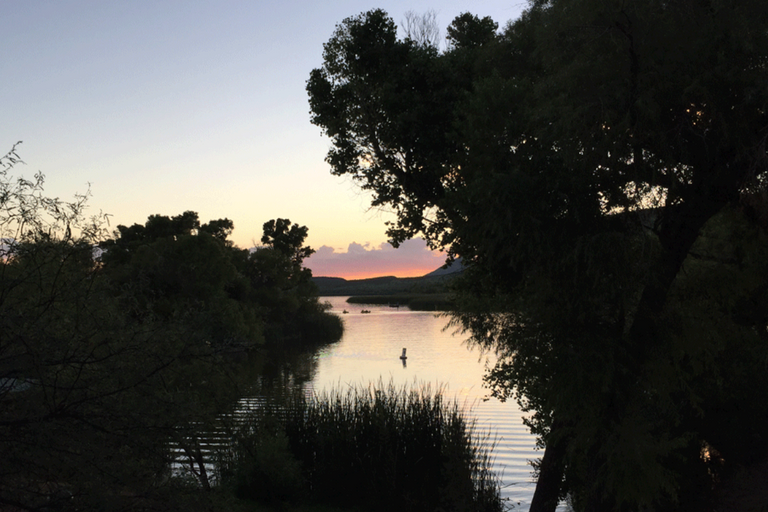This serene nature scene captures the calming transition of day to night over a tranquil body of water, likely a river or lake. The sun is setting, painting the sky with stunning hues of reddish-orange and pinkish-purple. Faint, wispy clouds catch the sun’s final rays, adding to the picturesque backdrop. The water’s surface is mostly calm, disturbed only by gentle ripples likely caused by a light breeze. In the middle of the water, a buoy or perhaps some birds are visible, accentuating the peacefulness. Surrounding the water are lush trees and dense shrubbery, which frame the scene beautifully. Tall grass juts into the water, further enhancing the natural, untouched feel of the landscape. To the right and left, tree cover extends into a backdrop of rolling hills or distant mountains, completing this idyllic sunset view.